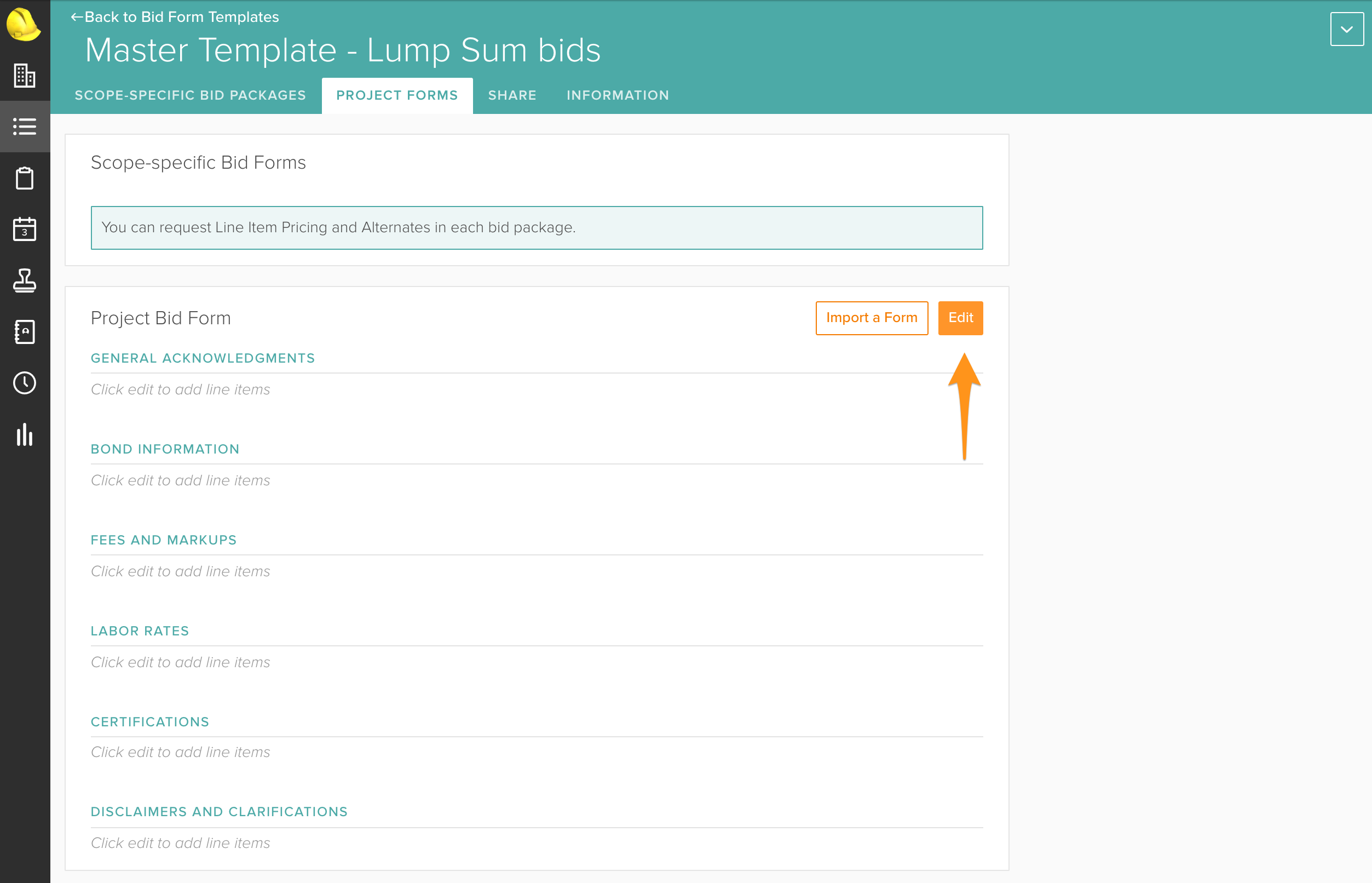The image displays an interface with a bluish-dark blue-greenish colored border, which features a header titled "Back to Bid Form Templates." Directly below the header is the subtitle "Master Template for Lump Sum Bids" accompanied by "Scope Specific Bid Packages" and "Project Forms to Share Information." 

Beneath that, the section is labeled "Scope Specific Bid Forms," followed by a light blue box containing instructions: "You can request line item pricing and alternates in each bid package."

On the right side of this section, there are two buttons: a white button labeled "Import a Form" and an orange button labeled "Edit." There is also a distinct orange arrow pointing directly at the "Edit" button.

To the left, there is a list of categories with corresponding prompts to add details:

1. "Project Bid Form General Acknowledgments" with a prompt "Click edit to add line items"
2. "Bond Information" with a prompt "Click edit to add line items"
3. "Fees and Markups" with a prompt "Click edit to add line items"
4. "Labor Rates" with a prompt "Click edit to add line items"

Each category includes the instruction "Click edit to add line items," inviting the user to input specific information.